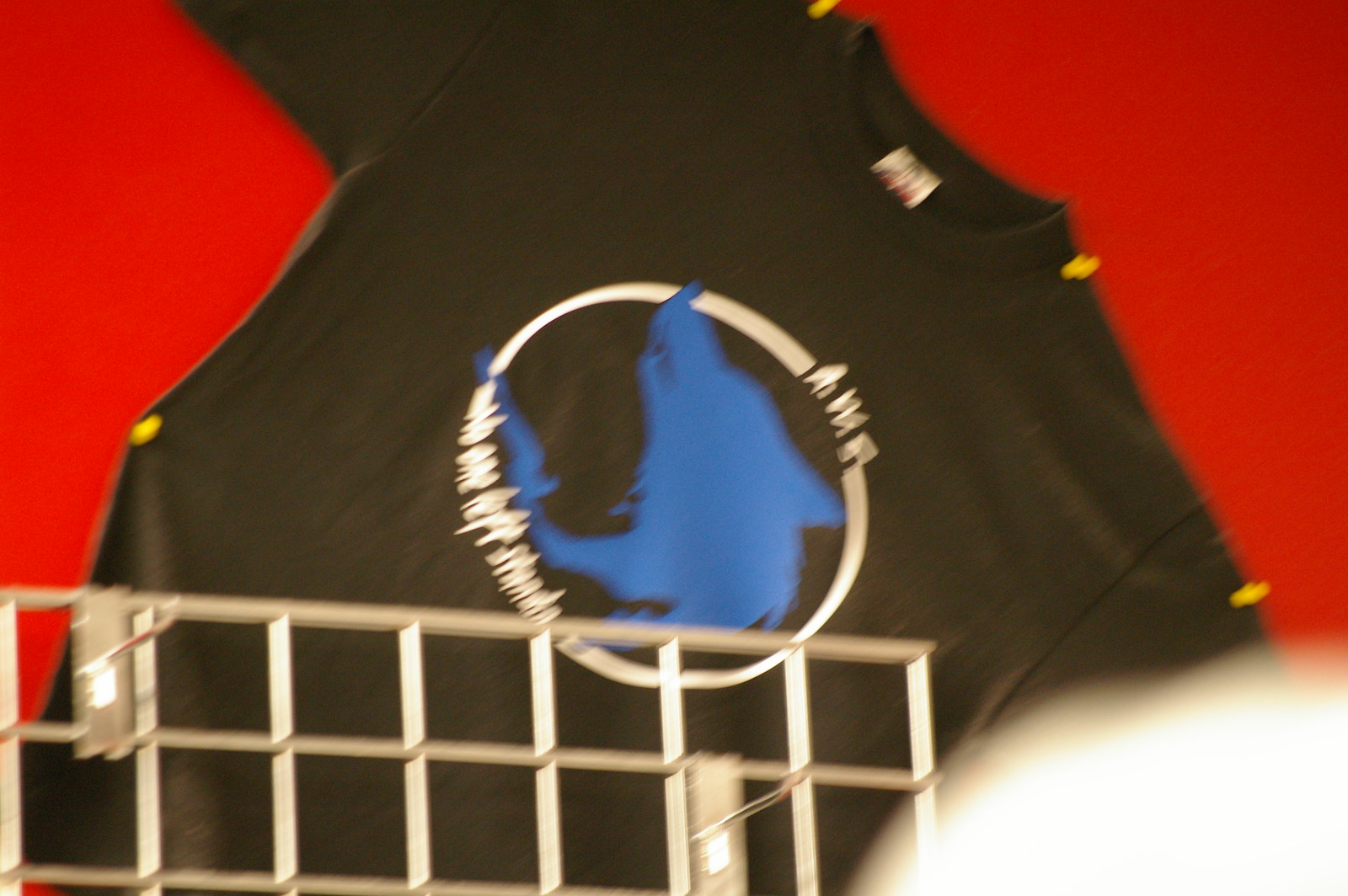This image showcases a black short-sleeved t-shirt pinned to a red background using yellow pushpins. The shirt features a prominent design in the center: a blue canine, possibly a shark or wolf, encapsulated within a white circle. Text is visible at the top and bottom of the circle, although it's illegible. The label of the t-shirt can be seen at the top near the collar. The image appears slightly angled, causing the right sleeve to extend towards the upper left corner and the left sleeve towards the bottom right. The photograph is tightly cropped around the t-shirt, with other materials visible in the peripheral areas. At the bottom right, the shoulder of a person wearing a white shirt is partially visible, and in the bottom left, a wire display rack with hooks can be discerned, suggesting a retail setting.